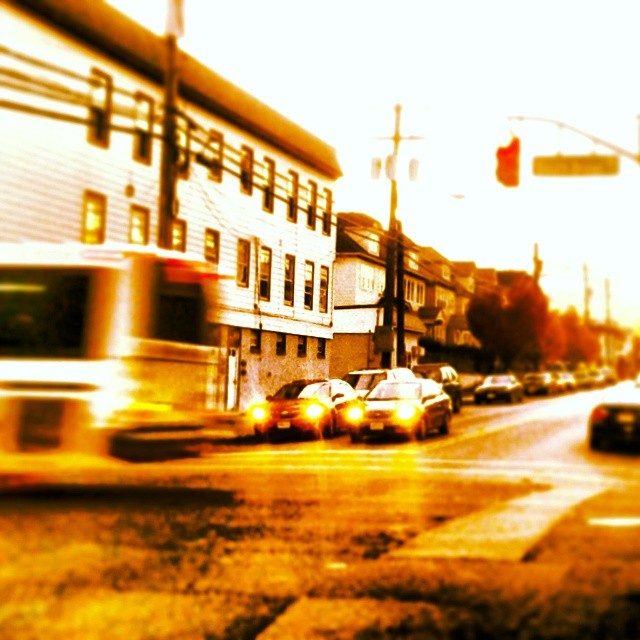This is an artistic, somewhat grainy photograph with a sepia tone filter, giving it a soft golden glow. It depicts a bustling city intersection with a horizontally running street occupying the lower third of the image. In the foreground, a streetlight and an overexposed street sign sit overhead, casting a bright glare. The tail end of a bus, blurred with motion, crosses the intersection from left to right. At the intersection, a car with its headlights on faces the bus, while to the left, another car with headlights on, appears to be red. Behind these cars, two SUVs are faintly visible, and numerous cars are parked along both sides of the street. Notable is a large building on the corner with 18 visible windows on the upper floors and four smaller windows below, along with a door. The building and the street are framed by trees and power lines that stretch down the street. The background is lined with what looks like residential dwellings and more parked cars, creating a vivid snapshot of urban life. Predominant colors in the photo include shades of white, gold, red, and black, adding to its vintage, yet dynamic feel.